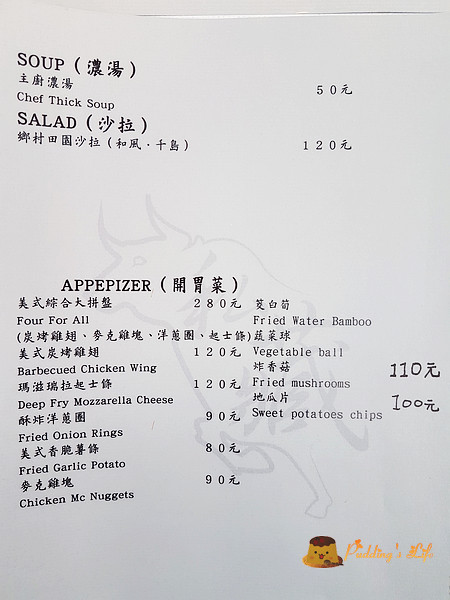Here is an image of a menu set against a white background in portrait orientation. The backdrop of the menu features a semi-transparent, pale gray illustration of a bowl. The menu text is layered on top of this background, starting from the top left corner. 

In black ink, with all capital letters, the first heading reads "SOUP," followed by Chinese characters in parentheses. Beneath this heading, additional Chinese characters are present. Below, in a mix of uppercase and lowercase letters, the item "Chef Thick Soup" is listed, priced at 50 units of an unspecified currency.

The next section, following the same format of all caps and parenthesized Chinese characters, reads "SALAD," and is priced at $1.20. 

Midway down the page, another heading reads "APPETIZER," accompanied by more Chinese characters. Detailed below are the following items along with their respective prices:
- Barbecued Chicken Wing: $2.80
- Deep Fried Mozzarella Cheese: $1.20
- Fried Onion Rings: $1.20
- Fried Garlic Potato: $1.90
- Chicken McNuggets: $1.80
- Fried Water Bamboo: $1.90
- Vegetable Ball: $1.10
- Fried Mushrooms: $1.00
- Sweet Potato Chips: $1.00

At the bottom of the menu, there is a whimsical cartoon illustration of a dessert with a smiling face. This depicts a gold-colored pudding topped with chocolate, accompanied by the caption, "Pudding's Life."